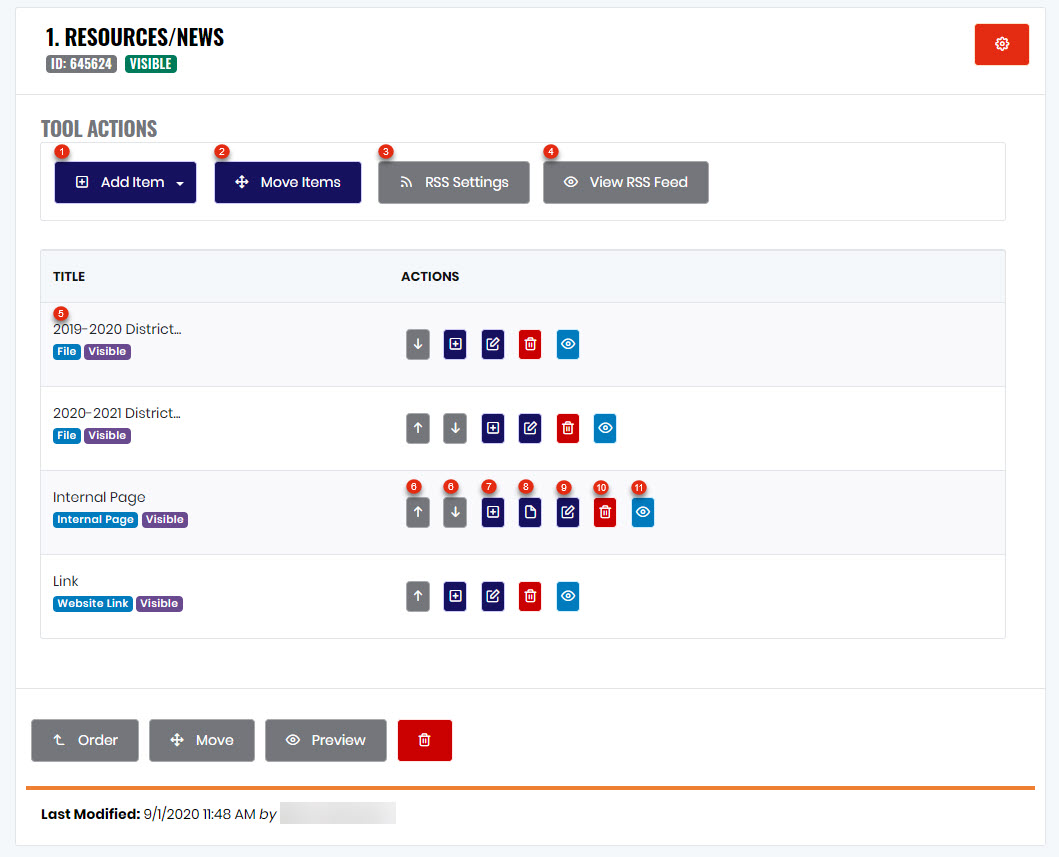This is a detailed caption for the image:

---

The image depicts a user interface loaded with various information and action options. In the upper left corner, "resources/news" is prominently displayed, accompanied by an ID number "6456" followed by a space. On the right corner, a settings icon in white sits within a red square. Below it is a horizontal gray line, followed by labeled tool actions: "Admit," "Add Item," "Move Items," "RSS Settings," and "View RSS Feed." Each action label features a red circle with a sequential number: "1" for Add Item, "2" for Move Items, "3" for RSS Settings, and "4" for View RSS Feed.

Underneath this section, there is a segment titled "Title Actions." Beneath this title, a list of four items is displayed, each accompanied by action options represented by icons:
1. The first item, marked with a circled "5", is titled "2019-2022 District File." It showcases a sequence of icons for various actions: a square icon with a plus sign for adding, an edit icon, a trash icon for deleting, and a view icon.
2. The second item, "2020-2021 District," follows with similar actions and includes options for uploading and downloading files.
3. The third line details an item named "Internal Page," equipped with the same action icons.
4. The fourth item lists several action icons marked with numbers "6" for upload, "7" for download, "8" for add, "9" for page, "10" for edit, "11" for trash, and "12" for visibility.

A comprehensive array of tools and actions is efficiently organized, allowing for detailed management and navigation.